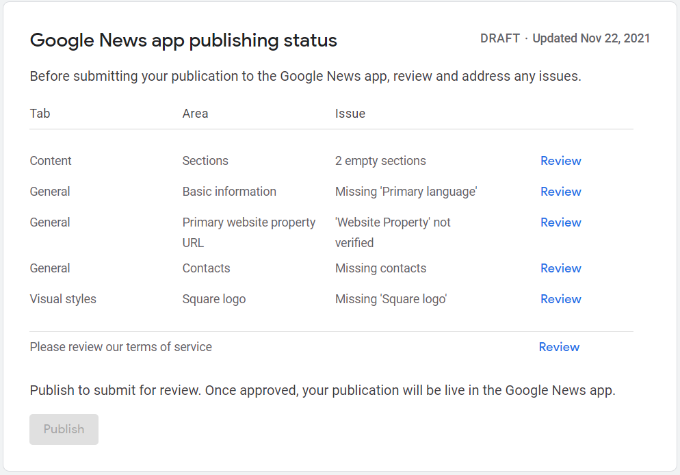This rectangular, panoramic image, bordered by thin gray lines, features a completely white interior. In the upper-left corner, the title "Google News App Publishing Status" is displayed in gray, upper-case letters, followed by "UPDATED: NOV 22, 2021" also in gray. Below the title is an advisory note: "Before submitting your publication to the Google News App, review and address any issues."

From left to right, the image is divided into three columns labeled "Tabs," "Area," and "Issue," with a thin gray bar below these headings. Under "Tabs," the entries, in order from top to bottom, are: "Content," "General," "General," "General," and "Visual Styles," all in gray letters. Under "Area," the corresponding entries are: "Sections," "Basic Information," "Primary Website Property URL," "Contact," and "Square Logo." Under "Issue," the listed problems are: two empty sections, "Missing Primary Language," "Website Property Not Verified," "Missing Contact," and "Missing Square Logo."

To the right of each issue is the word "Review" in blue letters. Below the listed tabs, areas, and issues is a faint gray line running horizontally across the image. On the lower left, there is a note: "Please review our terms of service," accompanied by another "Review" in blue on the far right. Beneath this section, a black sentence reads: "Publish to submit for review. Once approved, your publication will be live in the Google News App."

In the very lower-left corner is a gray button labeled "Publish," but it is grayed out, indicating it is currently unclickable.